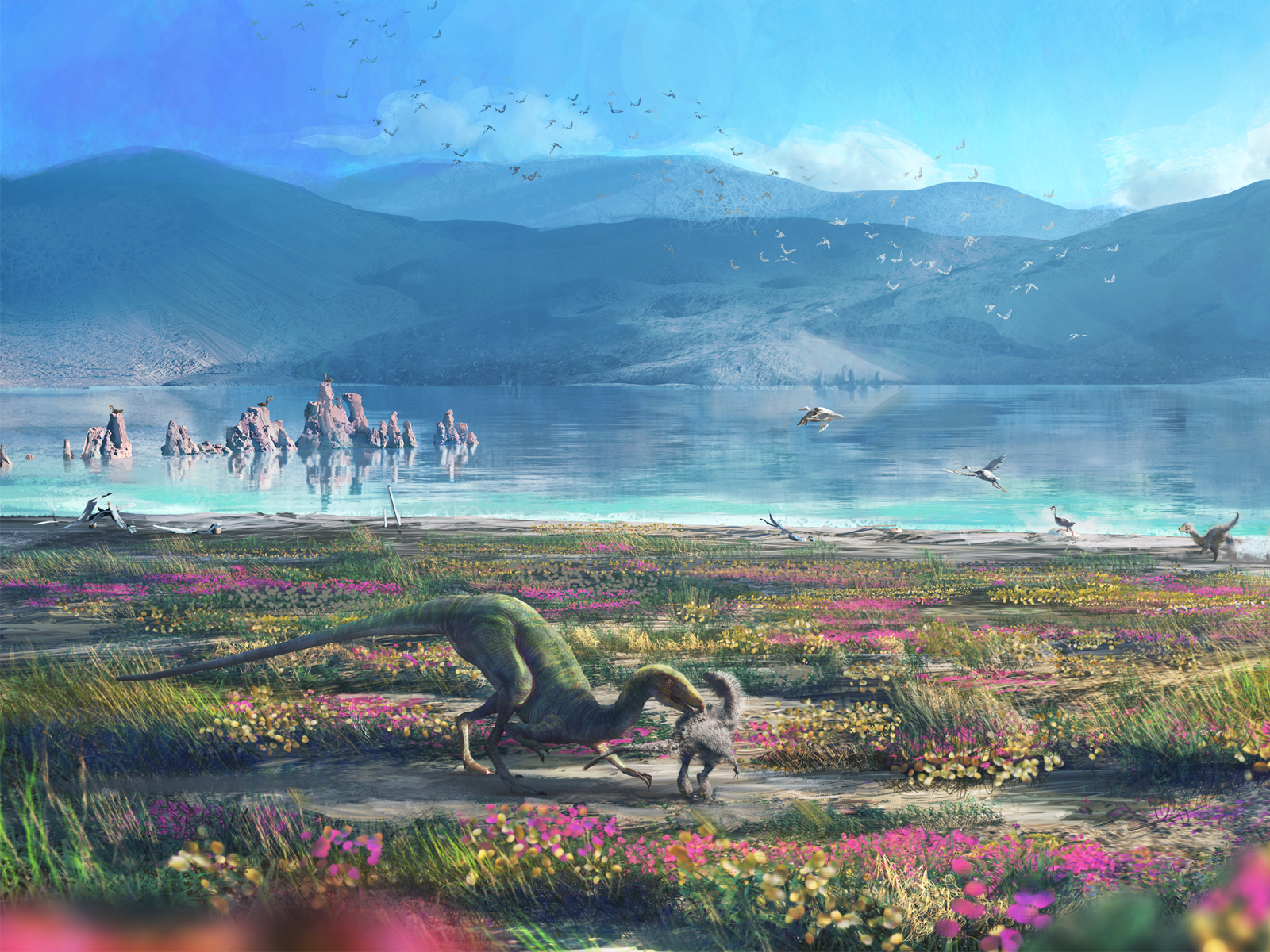This painting vividly depicts a prehistoric landscape teeming with life. Dominating the foreground is a green dinosaur with a yellow head, resembling a raptor. It is poised aggressively, mouth open, capturing or chewing on a smaller gray creature that looks like an ostrich or bird. Surrounding them is a lush field of green grass adorned with pink, yellow, and purple flowers, creating a vibrant and colorful scene. Further back, a large body of water, a huge lake with a mix of blue and teal hues, stretches across the lowlands. Birds, possibly ducks and seagulls, are seen cleaning themselves in the water, flying above it, and resting on rock formations that protrude from the lake. In the distance, a dramatic mountain range rises, adding depth to the scene. The sky above is a rich blue, scattered with gray clouds, completing the atmospheric backdrop of this striking and dynamic prehistoric setting.